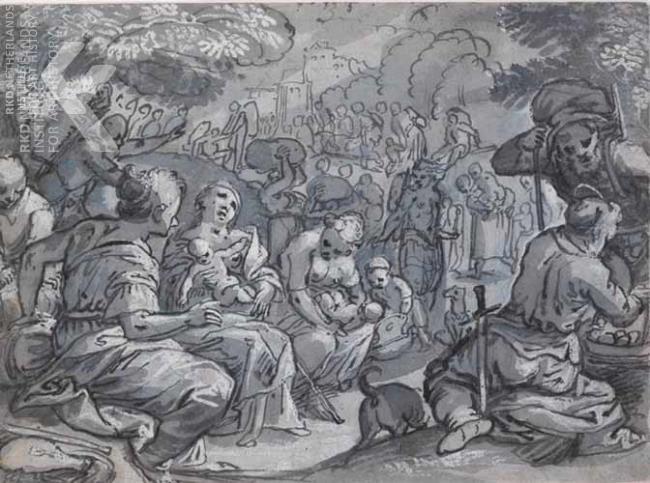The image is a detailed, black and white drawing, likely a painting still in progress, with a rectangular orientation. The scene is densely populated with numerous figures, emphasizing their emotional states through intricate detailing. In the foreground, on the left-hand side, several women are seated in a row, each appearing distressed, holding naked babies in their laps, with some women positioned behind them. A child and the back end of a dog can be seen among these figures.

On the right side of the image, a man with his back turned and partially in profile may be an artist or perhaps someone preparing the models. Near him, another man is kneeling, with a sword strapped to his waist, seemingly aiding an older man wearing a hat. Additionally, a person carrying a sack over their shoulder is visible on this side, further adding to the narrative depth.

The composition's background includes loosely sketched buildings and swirling lines that suggest trees. Partial and faint letters are discernible in the top left corner, adding an enigmatic element. Overall, the grayscale tones and artistic rendering highlight the emotional gravity and complex interactions of the scene.